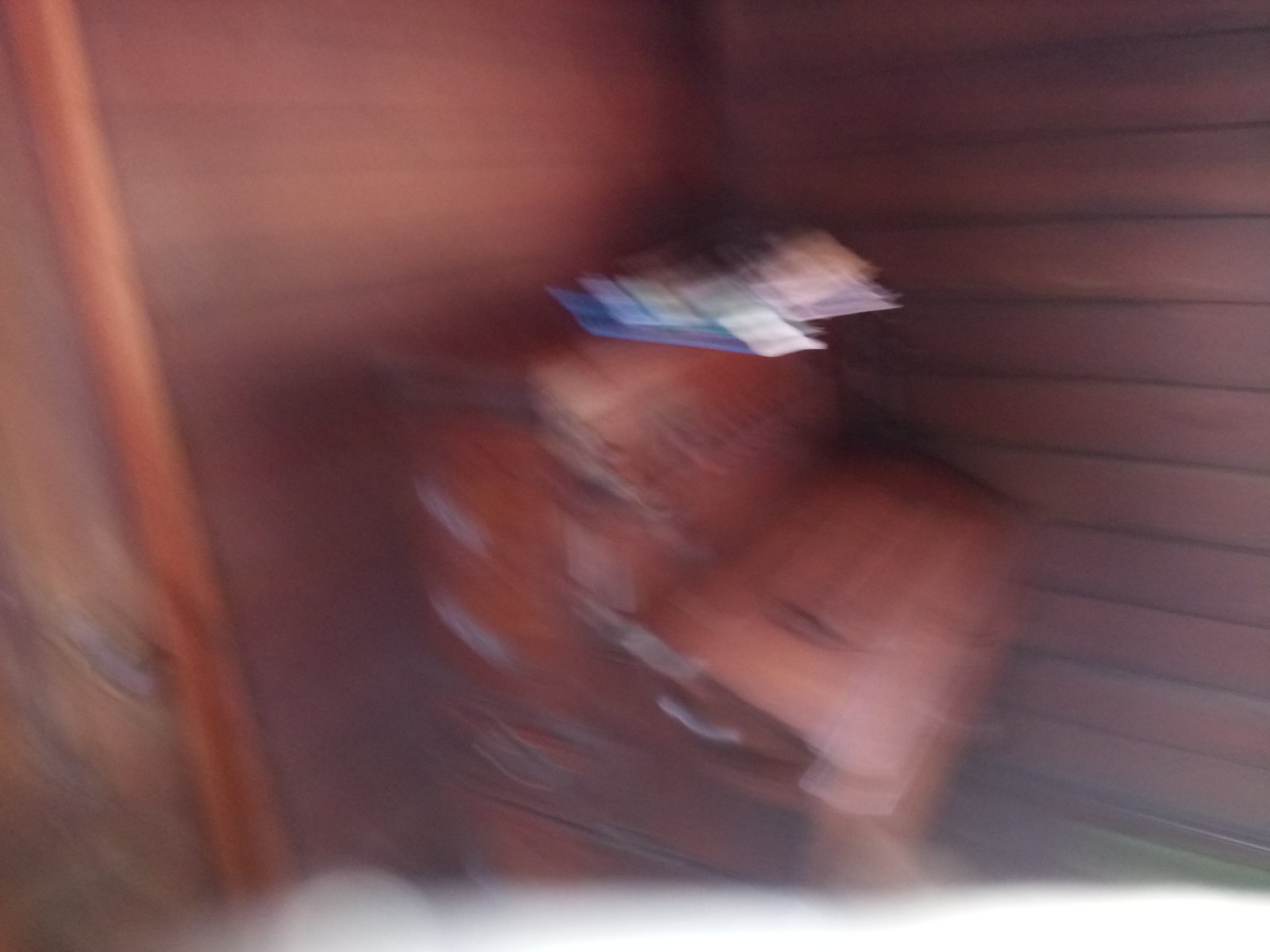The image depicts an indoor setting with a predominantly brown background wall, extending towards the right side of the frame. In the foreground, there is a wooden desk with distinct wooden grain patterns, although the shot is somewhat blurry. Behind the desk, the background includes various wooden elements. On top of the desk, there are scattered papers and what appears to be a piano, partially visible amidst the clutter. The overall atmosphere gives a warm, rustic impression, enhanced by the rich brown tones and wooden textures throughout the scene.